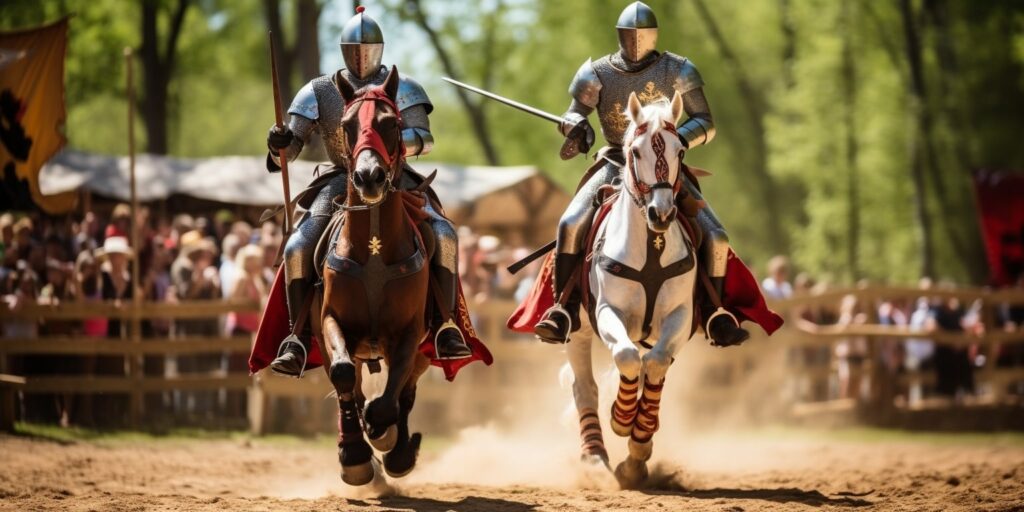In the image, two armored knights are galloping towards the camera on horseback, possibly part of a jousting event or a Renaissance festival. The knight on the right rides a white horse adorned with a distinctive brown strap across its chest and a red strap down its forehead. The horse features yellow and red striped wraps around its ankles. The knight is clad in silver armor with a chrome-colored face mask, holding a sword in his left hand while his feet rest in silver-colored stirrups.

To the left, the other knight rides a brown horse decorated with a red mask-like cover and a dark black chest strap. This knight, also dressed in reflective silver armor, wears a red coat, with his feet securely in silver-colored stirrups. His horse is in mid-gallop, nearly having all feet off the ground. Both knights appear to be participating in a jousting match, with the one on the right holding a sword and the one on the left possibly wielding a lance.

In the background, a blurred crowd gathers behind split-rail fences, suggesting an audience engrossed in the event. The scene is set against a lush green forest and a structure resembling a park pavilion. The overall atmosphere evokes a festival or a medieval-themed movie, highlighted by the spectators' attire and the knights' detailed armor.